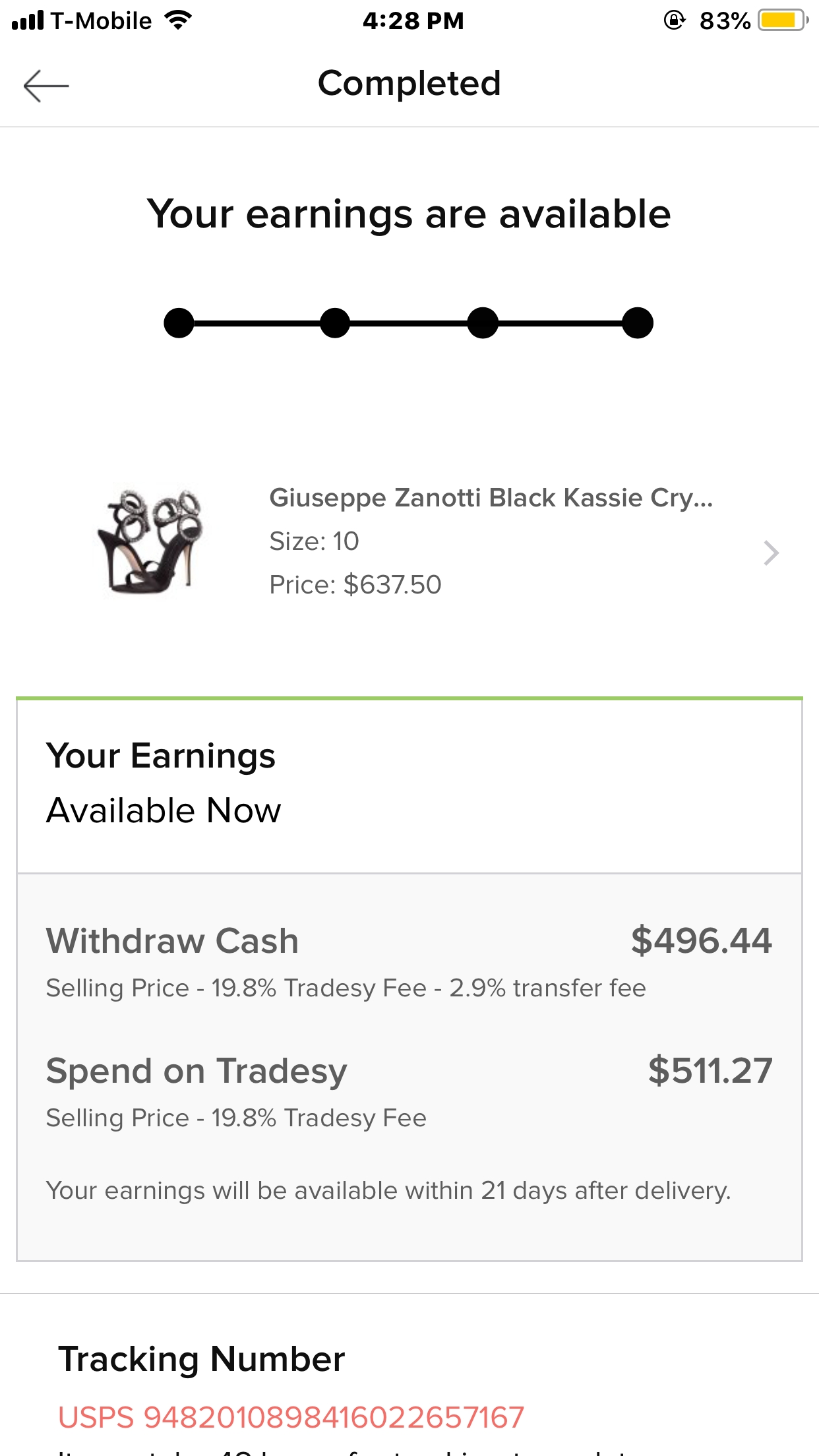The image depicts a smartphone screen showcasing a detailed status update on a sale made via the Trade Z app. At the top, the status bar reveals it is 4:28 p.m. with a full T-Mobile cell service signal and a strong Wi-Fi connection. The phone's battery is at 83%, displayed in yellow, indicating low power mode is on. The device orientation is locked.

The primary screen content is predominantly black and white, with occasional splashes of color. The header features the word "Completed" in black, verifying the transaction status. To the left, a back arrow icon provides navigation to the previous screen. Below, a notification states "Your earnings are available," followed by a decorative sequence of dots and lines.

Central to the image is a prominently displayed photograph of a pair of high-heeled stilettos, specifically the Giuseppe Zanotti Black Cassie Cry in size 10, priced at $637.50. Adjacent to the image is a gray box containing details about the seller's available earnings. It explains the breakdown of the final price: a 19.8% selling fee, a 2.9% Trade Z fee, and associated transfer costs, culminating in a net earnings figure of $496.44.

Additionally, the box provides an option to reinvest the earnings on Trade Z, specifying a net figure of $511.27 after excluding the selling and Trade Z fees. The caption confirms that these earnings will be available within 21 days post-delivery. At the bottom, a tracking number for USPS, highlighted in red, is provided for item location and status monitoring.